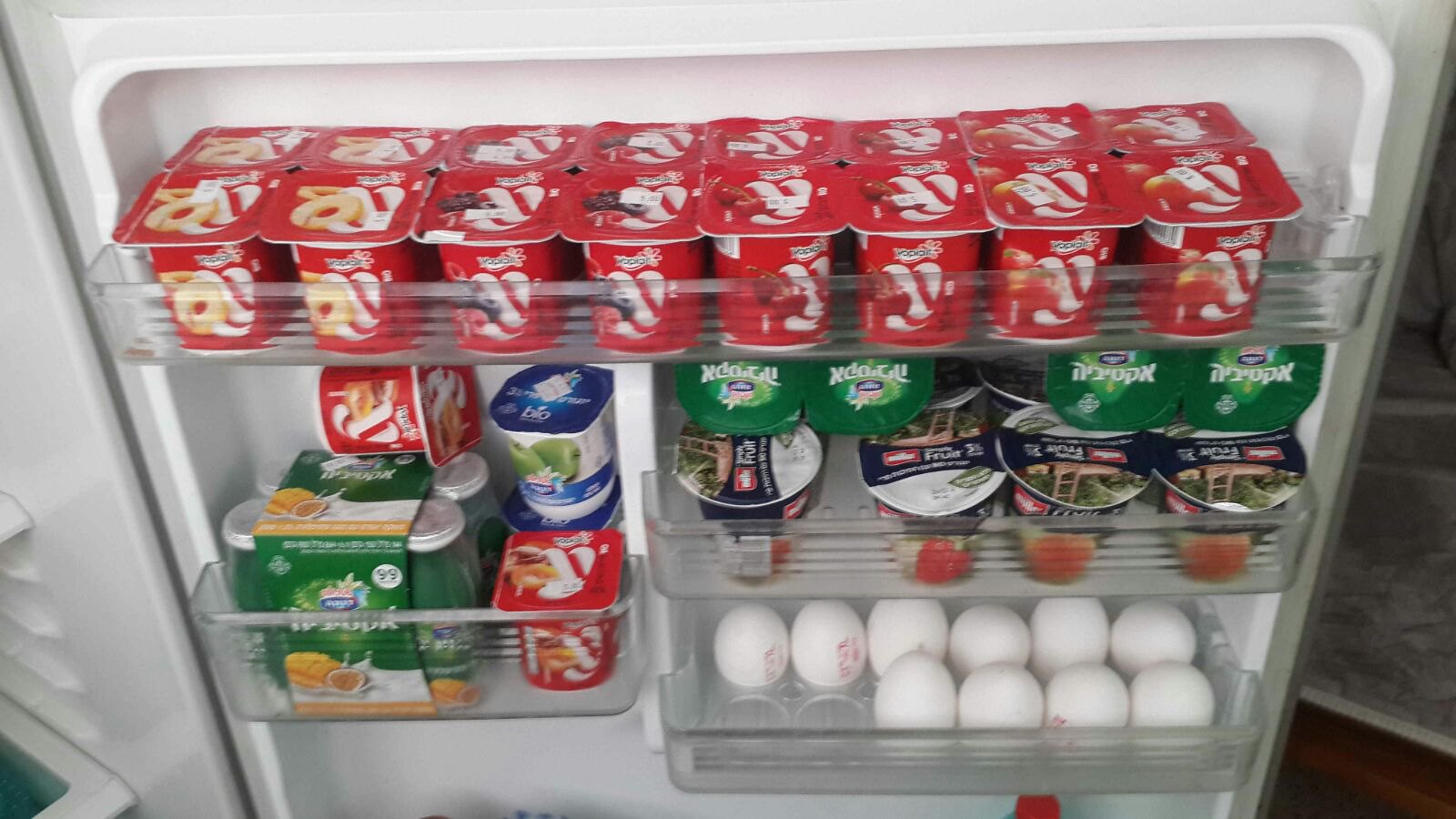This photograph depicts the inside of an open white refrigerator door. The top shelf is packed with over a dozen red Yoplait yogurt cups, arranged in neat rows, including flavors such as peach, mixed berry, cherry, and possibly strawberry. Below the Yoplait yogurts, there are various other yogurt cups: some green with characters on them, indicating they may be from a different country, interspersed with blue and white packs. Further down, a drawer containing a container of white eggs is visible, with approximately ten eggs, some marked with red letters. The image, though blurry and of low quality, also provides a glimpse of a wood floor and a white or pink carpet on the right side of the background.